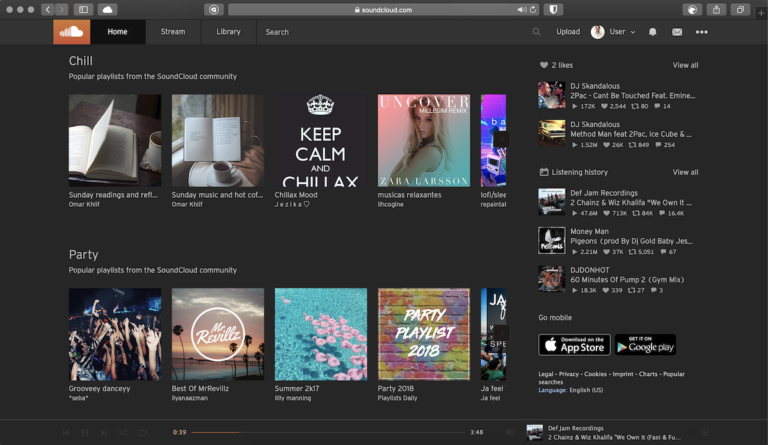On this page, we are viewing SoundCloud's interface, which features a sleek, completely black background. In the top left corner, we see the SoundCloud logo, a distinctive design of a cloud split in half: the left side is made up of horizontal white stripes while the right side is a solid white half against an orange backdrop.

Displayed prominently are playlists curated by the SoundCloud community, categorized as "chill" and "party" music. The "Chill" section includes the following:

1. **Sunday Readings** - A playlist designed for a relaxed Sunday vibe.
2. **Sunday Music and Hot Coffee** - Ideal for a serene, coffee-filled morning.
3. **Chillax Mood** - Featuring an album cover with a crown and the text "Keep Calm and Chillax."
4. **Musica Relaxantes** - Showcasing an album cover with a blonde woman, artist Zara Larson, exposing her left shoulder.

Next, we have the "Party" music section, also tagged as popular playlists by the SoundCloud community:

1. **Groovy Dancey** - A collection of upbeat tracks perfect for dancing.
2. **Best of Mr. Rebels** - A playlist featuring the top tracks by the artist Mr. Rebels.
3. **Summer 2k17** - Capturing the essence of summer with vibrant tunes from that year.